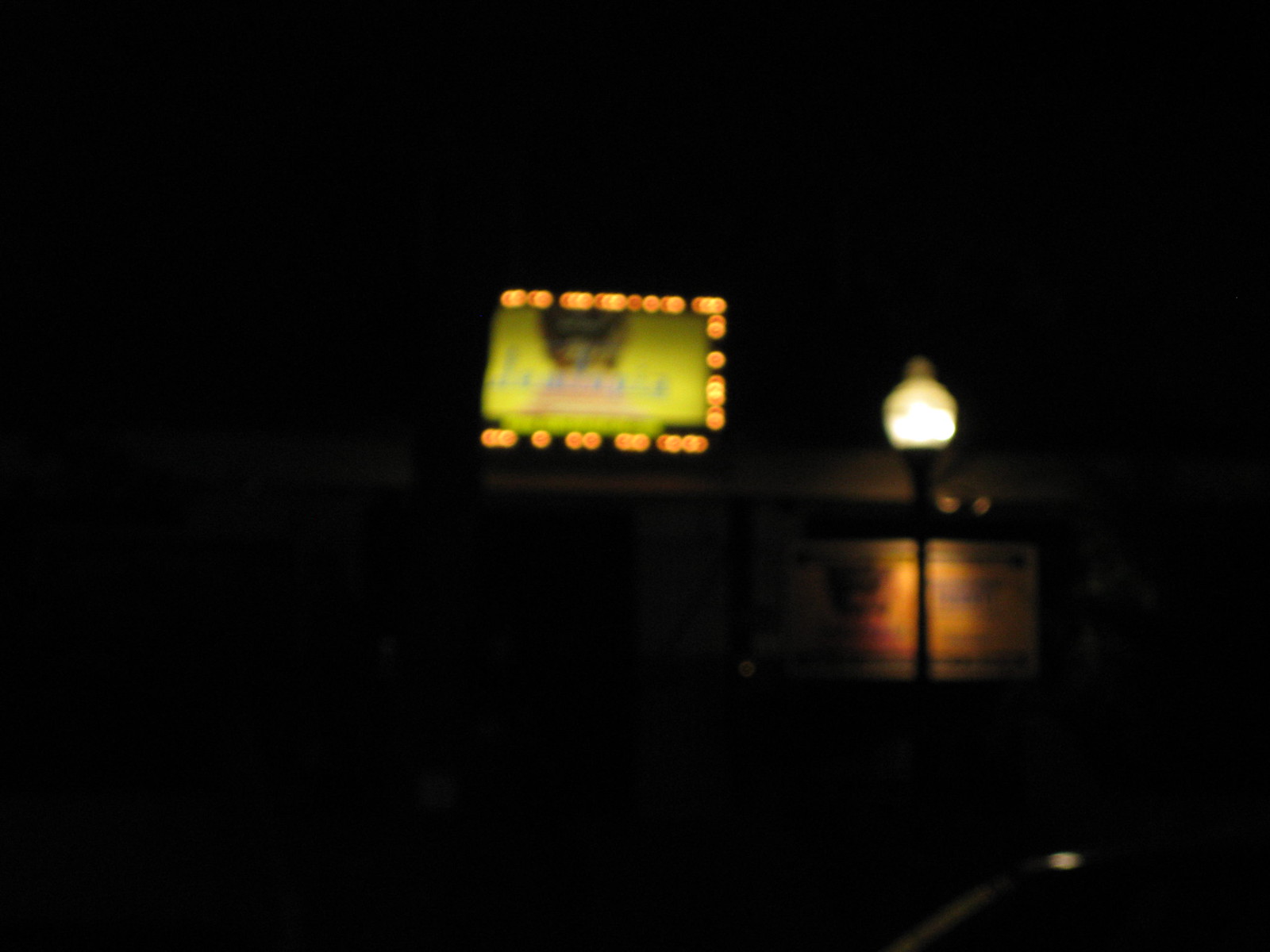The image depicts a somewhat blurred nighttime scene, likely taken on a road. The focal point of the photograph is a large billboard, possibly yellow in color, adorned with bright gold or yellow lights outlining its frame. The billboard features some form of cursive writing, though the text is indistinct due to the blur. Positioned in front of the billboard is a distinctive streetlamp with a spherical light and a rounded top, mounted on a black metal pole. Behind the streetlamp, there appears to be wooden structures, possibly chairs or another type of furniture. In the background, a few scattered lights dot the scene, suggesting it is evening. The overall ambiance is dimly lit, with the primary sources of illumination being the billboard and the streetlamp.